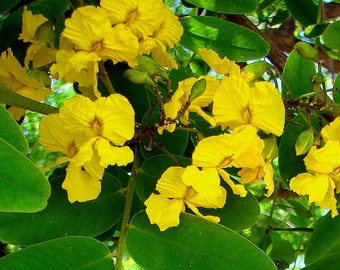This photograph, taken outdoors during a sunny day, captures a scene viewed upward through a canopy of tree leaves, with patches of blue sky visible between them. The image, though small and slightly pixelated at about 2 by 1.5 inches, reveals intricate details. In the upper right corner, brown branches are adorned with thick green vines bearing large, waxy, oval leaves that frame the scene. Clusters of delicate yellow flowers, each featuring 2 to 4 frilled petals, hang from the vines. These petals, gently wrinkled, are adorned with a central triangular or diamond-shaped dark orange or reddish marking. The interplay of light and shadow suggests a dappled effect, further enhancing the photograph's natural beauty. Despite its low resolution, the image's vivid elements and serene ambiance are palpable.